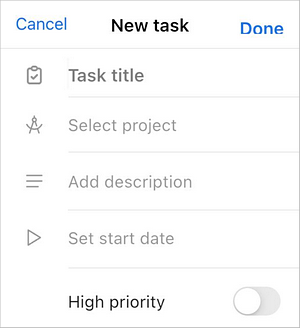Certainly! Here is the cleaned-up, detailed caption for the image described:

---

*Screenshot of a Task Management Interface*

The screenshot displays a task management interface on a person's phone with a clean white background. At the top, there is an upper banner with three options: "Cancel" (with a capital 'C'), "New Task," and "Done" (with a capital 'D'). Below the banner, there are various fields and icons to detail the task.

1. **Task Title:** This section features a grey clipboard icon with a piece of paper and a grey checkmark, indicating where the user can input the task title.
2. **Add Description:** Right underneath, there is a picture resembling a metal compass—suggesting precision and detail—accompanied by the text "add description" (with a capital 'A').
3. **Start Date:** The next item shows three horizontally stacked bars with the text "Start Date" (with a capital 'S'). 
4. **Priority Setting:** Following this, there is an option labeled "High Priority" (with a capital 'H'). This line includes a blue slider that has not been selected and is positioned to the left, indicating that the "High Priority" status is currently toggled off.

The interface’s dividing lines between each section are colored light grey, maintaining a minimalist design aesthetic against the white background.